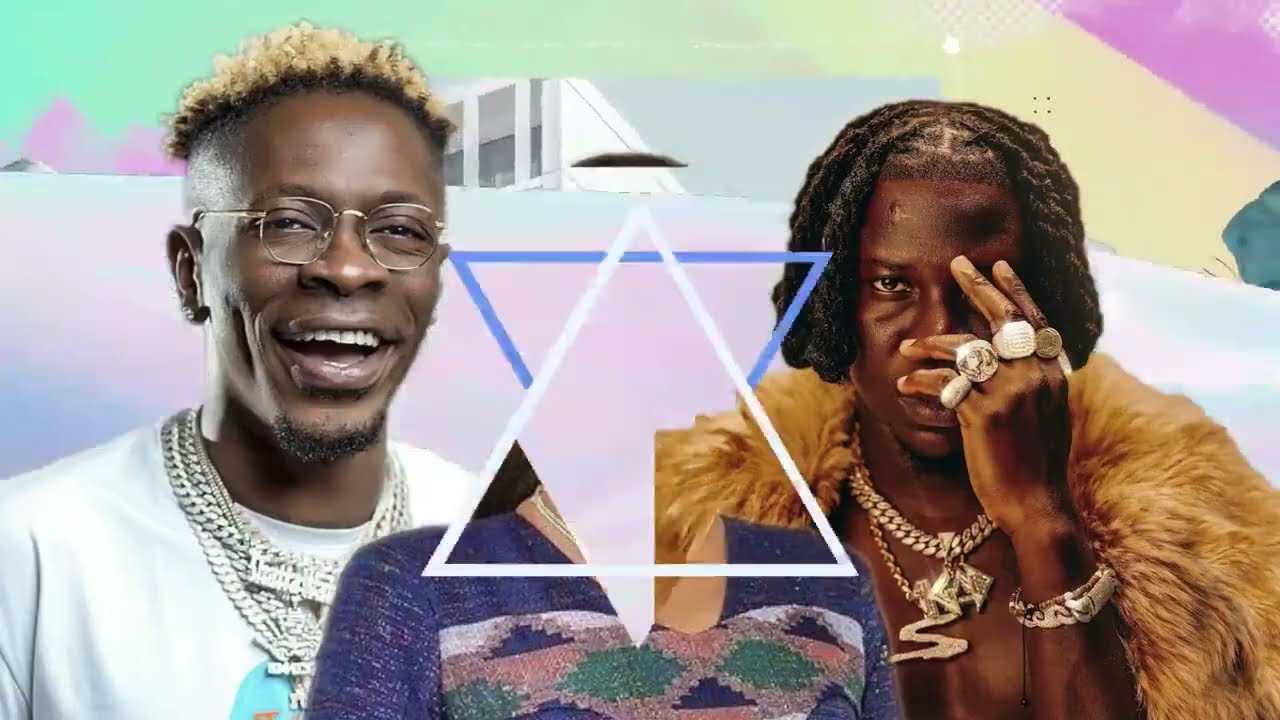The horizontal rectangular image depicts two Black individuals possibly engaged in a podcast or featured in a collage photograph, set against a dynamic and colorful background. On the left, a congenial Black man with cropped blonde-tipped hair and glasses is smiling warmly. He sports a white T-shirt adorned with multiple layers of silver chains and earrings, and a light beard. In the center, partially covering a figure in a cashmere-patterned sweater, is an enigmatic, white and blue Star of David. On the right, another Black individual, whose gender is not entirely discernible, exudes a more intense demeanor. They are clad in a beige fur cape, with their face partly obscured by a hand adorned with numerous gold rings. Gold jewelry, including a prominent bracelet and a large 'F' pendant necklace, further accessorizes their look. Their hair, styled in dreads falling just short of the shoulders, adds to their distinctive appearance. The background of the image is a tapestry of pastel hues: a whitish pink separates the two individuals, while above, a background transitions from teal-green with purple accents on the right to shades of pink and green. The overall composition, featuring abstract elements like a partially obscured building shape and horizon-like pastel graphics, injects a surreal and enigmatic quality into the image.